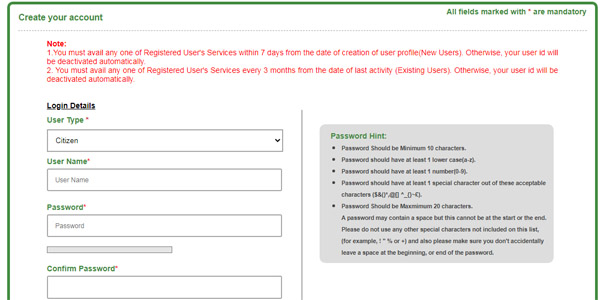The image features a user registration form set against a white background. At the top in green text, it reads "Create Your Account." The form highlights that all fields marked with a red asterisk (*) are mandatory. A note on the form specifies, "You must avail any one of the registered users' services within seven days from the date of creation of your user profile (for new users). Otherwise, your user ID will be deactivated automatically. Additionally, you must avail any one of the registered users' services every three months from the date of last activity (for existing users). Otherwise, your user ID will be deactivated automatically."

Below this note, the form includes the following sections:
- **Login Details:** 
  - **User Type:** Marked with a red asterisk, displaying a dropdown box with options like "Citizen."
  - **Username:** Also marked with a red asterisk, accompanied by an input box.
  - **Password:** Marked with a red asterisk, featuring an input box.
  - **Confirm Password:** Following the password field, another input box is provided.
  - To the right of the confirm password box, there is a gray square that contains "Password Hint" in green text.

A bulleted list provides password requirements:
- Password should be a minimum of 10 characters.
- Password must include at least one lowercase letter, specified as 'a' to 'r' in parentheses.